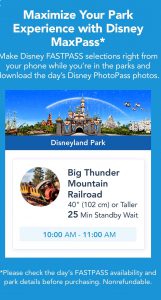**Enhance Your Park Experience with Disney MaxPass**

Set against a vibrant blue backdrop with white lettering, this advertisement invites visitors to maximize their Disneyland Park visit with Disney MaxPass.* At the top, the message reads, "Maximize your park experience with Disney MaxPass*," encouraging guests to make Disney FastPass selections directly from their phones and download daily Disney PhotoPass photos while exploring the park.

Contained within the main advertisement is a highlighted section featuring an illustration of the iconic Disney Castle under a bright blue, starry sky, with what appears to be a shooting star streaking behind it. Below this enchanting depiction, the text reads "Disneyland Park." Further below, guests can see a visual of the park entrance leading up to the castle.

In the lower part of this segment, a white square features a circle with an image of a train inside, which pertains to the Big Thunder Mountain Railroad attraction. It specifies that the ride requires a height of 40 inches or taller and currently has a standby wait time of 25 minutes, with availability from 10 a.m. to 11 a.m.

*Please note that the MaxPass service includes additional features and benefits which can be accessed from your mobile device.